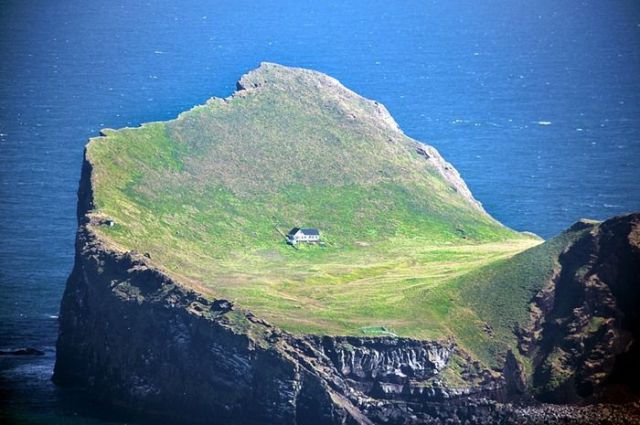This aerial photograph captures a dramatic and isolated land formation that appears to be either a peninsula or an island jutting out into a blue ocean. The central feature is a high, rugged rock formation covered with patches of green grass. It rises sharply from the sea and is reminiscent of a mountain sliced in half, with uneven, jagged edges and a low center flanked by higher cliffs. 

Atop this elevated, cliff-like land is a modest, solitary white house, standing out against the natural backdrop. The house, positioned in the middle of the formation, suggests it is either a private retreat or an isolated residence. The photo prominently displays the ocean to the left and top edges, emphasizing the land's seclusion and contrast against the vast expanse of water. The scene is devoid of any visible roads or pathways, adding to its remote and untouched charm. The colors in the image are predominantly blue, green, brown, yellow, gray, and black, capturing the natural hues of the ocean, rock, and vegetation under what appears to be midday sunlight. This striking visual hinting at a potential location in Eastern Canada, perfectly centered with nature at its most raw and captivating.